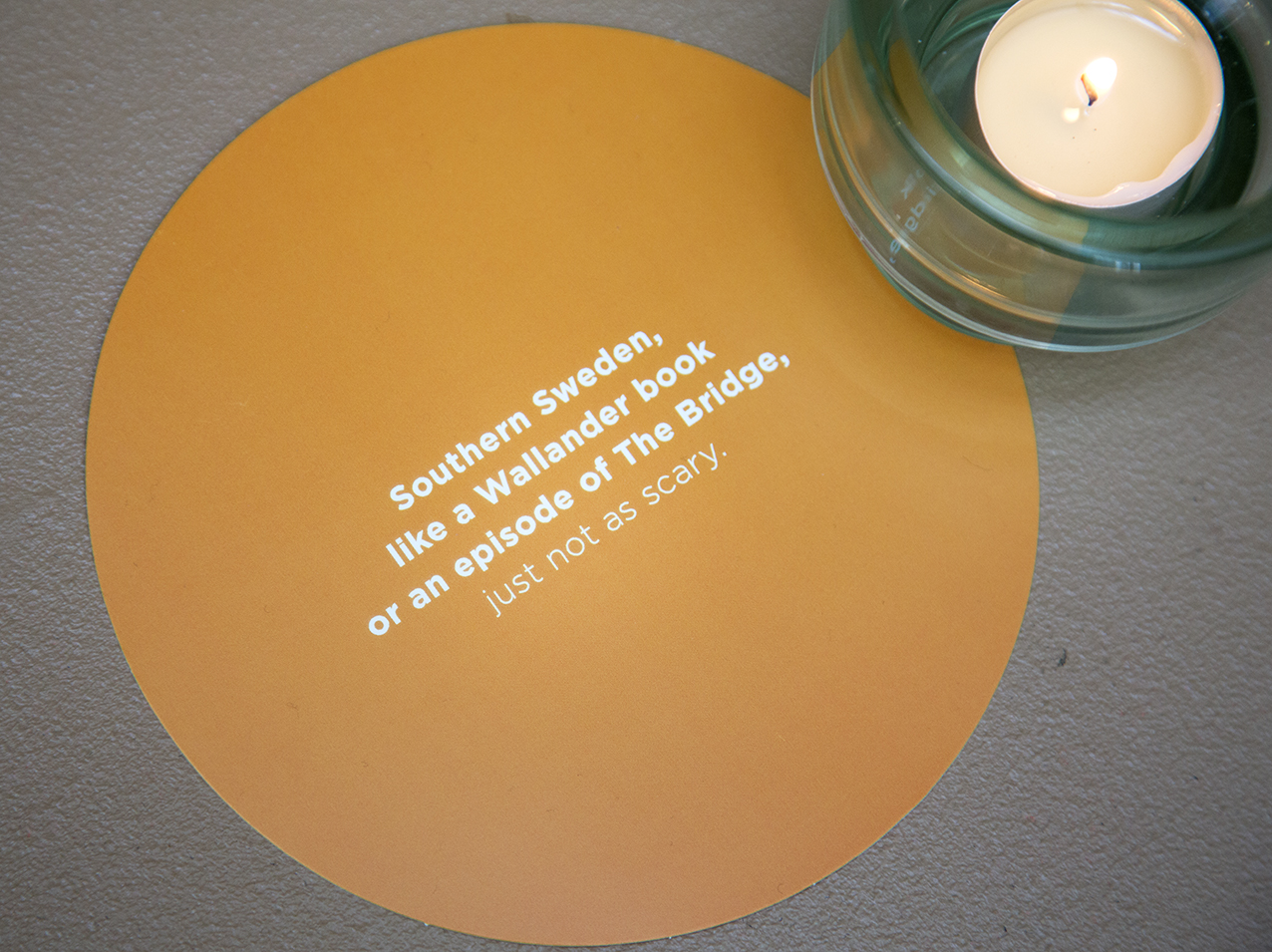On a hard, gray surface, possibly a tabletop, lies a round, bright orange piece of paper with white, angled text comprising four lines: "Southern Sweden," "Like a Wallander book," "Or an episode of The Bridge," "Just not as scary." Beside it, in the upper right-hand corner, a lit, creamy-colored candle is nestled in a clear, round glass holder, partially extending off the top and right edges of the image. The stark white text on the orange circle, along with the glowing candle, creates a vivid contrast against the minimalist background.